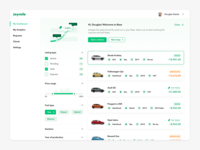The image appears to be a screenshot of a car shopping website. Dominating the center of the screen are various vehicles displayed in a grid format. Each vehicle showcases a different color, including silver, yellow, larger-sized vehicle, orange, red, and blue, all uniformly facing the same direction. Beneath each vehicle are four distinct facts or features, providing key information to easily compare each model, though they are not arranged in a tabular format.

On the right side of the screen, there appears to be contact information or options for reaching out to a representative. Central to the screen is a menu that offers customization or filtering choices; three selections have been highlighted or chosen in this section. To the far left is a smaller navigation menu, likely providing links to main sections such as car listings, purchasing options, or other related pages. Overall, the interface is designed to facilitate an easy comparison of vehicle features, menus for customization, contact information, and navigational aids.